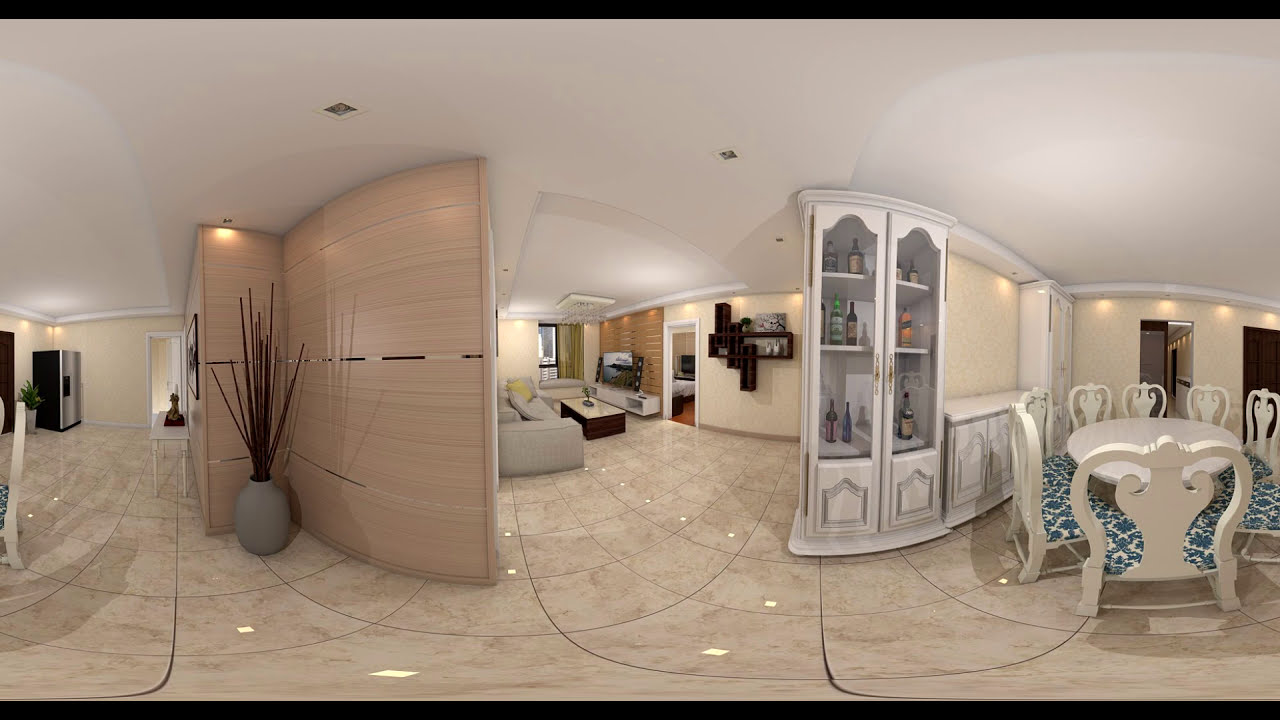This image is a panoramic shot of a lavish, photorealistically rendered home interior, exhibiting both photographic realism and subtle signs of animation. The flooring is polished brown marble tiles with reflections of ceiling lights enhancing its sheen. On the far left, the scene begins with a large gray planter containing vertical brown sticks, adjacent to a black and silver refrigerator. 

Toward the center left, a yellow accent wall borders another space showcasing a grand gray couch arranged around a white console with a TV. The TV cabinet, made of brown wood, is flanked by two vertical speakers and features a green curtain-covered window behind it. To the right of this entertainment area, a large window with open curtains bathes the room in natural light. 

In the central part of the image, a pseudo doorway leads to a larger room characterized by similar yellow-colored walls, comfortable gray couches, and a brown table with a glass top adorned by flower vases. Above, a designer light hangs from a white ceiling enhanced with a decorative false ceiling.

Just to the right of this setup is a distinct white dining area featuring an eight-seater round table encircled by white chairs patterned with blue and white floral designs. This dining space is flanked by a white china cabinet with transparent glass doors displaying an assortment of drinks and other items. Behind this area, a sleek kitchen is partially visible, crowded with various equipment.

On the far right of the panorama, another entryway seems to lead into a bedroom with a white bed and a side table. Overall, the area is well-lit, and the design elements like accent walls, designer lights, and various cabinets contribute to a high-end, welcoming atmosphere.